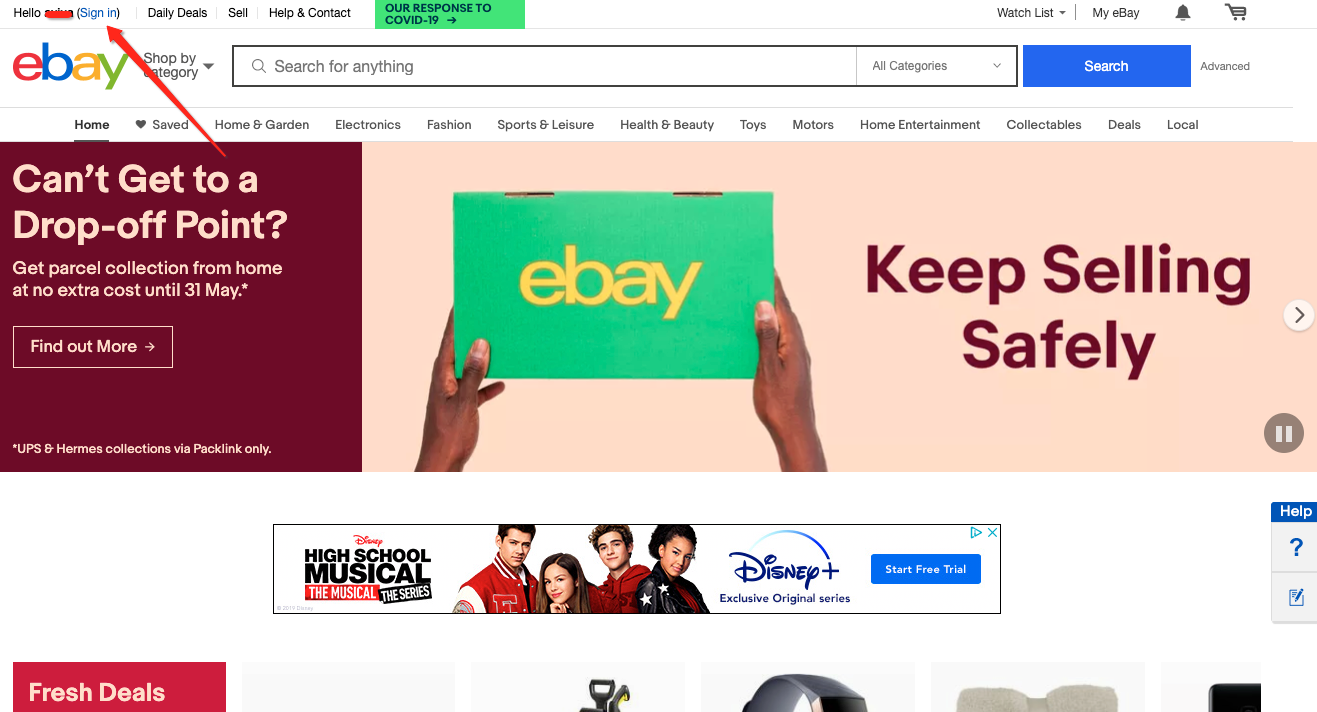In this image, we see the homepage of eBay, featuring its iconic multicolored logo in red, blue, yellow, and green positioned at the top left. An arrow points toward the "Sign In" button on the top right of the screen. Various navigation links are displayed, including "Shop by category," "Daily Deals," "Sell," "Help," and "Contact." A prominent banner at the top also addresses "Our response to COVID-19."

The search bar is prominently placed at the center, allowing users to enter keywords to "Save, search for anything." Additional options to the right of the search bar include the "Watch List," "My eBay," a notification bell icon, and the shopping cart icon.

A highlighted promotional message is visible, informing users that they can "Get parcel collection from home at no extra cost until the 31st of May," with an invitation to "Find out more." The text on the webpage is presented in a variety of colors, including green, yellow, red, pink, black, and white, adding to the visual appeal and differentiation of information.